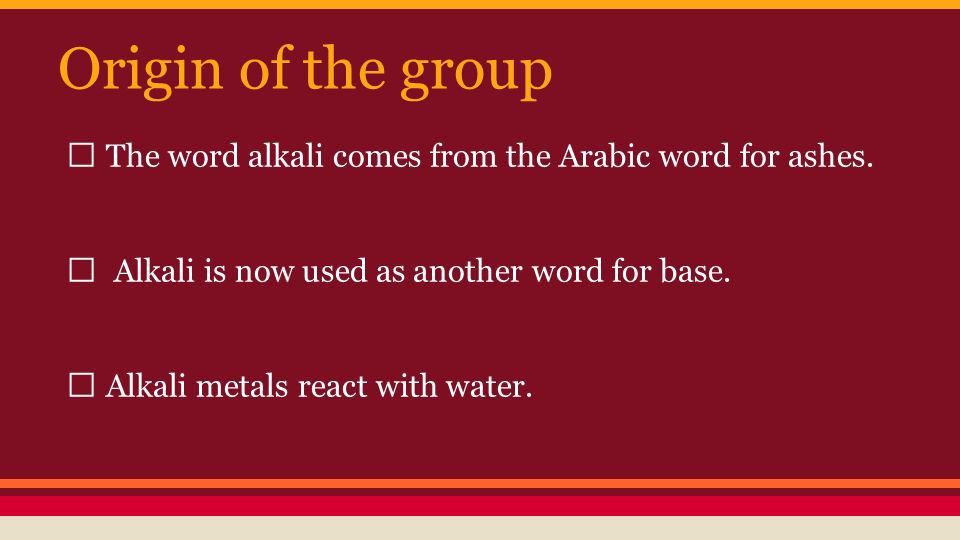The image features a text layout that resembles an index card set against a deep purple background. Across the top, there's a narrow yellow stripe, beneath which the title "Origin of the Group" is prominently displayed in large orange Cambria font. The text is organized into three detailed bullet points, each marked by white square outlines. The first bullet point states that "the word alkali comes from the Arabic word for ashes," while the second explains that "alkali is now used as another word for base." The third bullet point notes that "alkali metals react with water." Following these points, the bottom of the image is bordered by a series of colorful stripes: a dark orange line, a maroon strip, a bright red strip, and a final cream-colored strip.